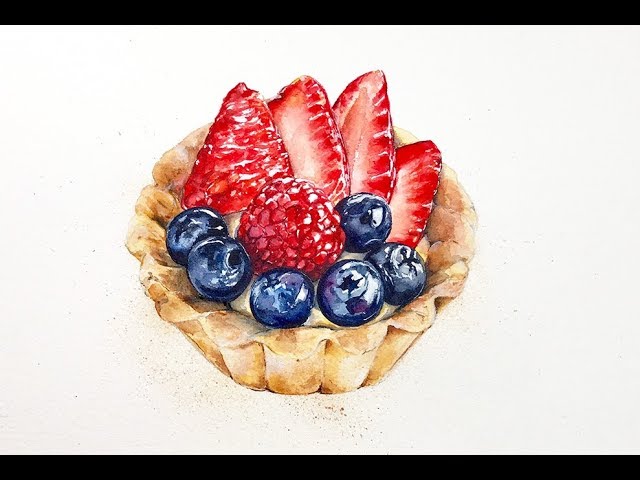This horizontal rectangle painting, a detailed and realistic modern artwork created in the last 50 years, showcases a delectable fruit tart. The tart, which occupies around 60% of the frame, sits at the center and is viewed from above. It rests in a fluted, light brown pastry cup, its color indicating it has been baked. The cup sits on a white surface with some visible discoloration, possibly due to the painting's age. Inside, a creamy, light-colored custard or cream filling forms the base. 

Arranged meticulously on top, a single red raspberry is positioned centrally, surrounded by six plump blueberries near the front edge of the tart. Four halved strawberry slices, vibrant red and fresh-looking, are positioned towards the back. Crumbs are scattered around the tart's base, adding an additional touch of realism. The painting's background remains an unadorned white, bounded by two horizontal black stripes at the top and bottom edges. The artist's skillful use of light reflections and careful attention to detail render the fruit and textures lifelike and appetizing. The colors of the fruits and pastry crust are vividly captured, making the tart look enticingly real.